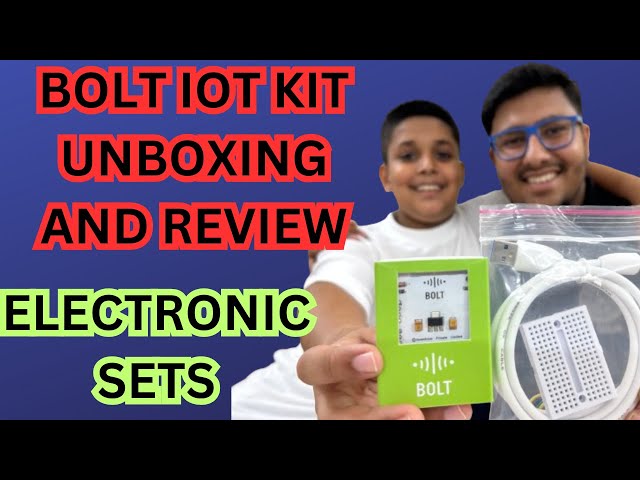The image is a highly detailed, computer-generated screenshot, seemingly from a YouTube video or blog post meant to review an electronic product. The background is a dark navy blue with noticeable thick black bars at the top and bottom, framing the central content. On the left side of the image, bold text reads "Bolt IoT Kit Unboxing and Review" in black with a red outline, and below it, "Electronic Sets" in black with a neon green outline.

On the right side, two young males are featured, both with brown complexions and black hair, potentially of Indian descent. The younger individual, around 17 years old, is dressed in a white T-shirt and is smiling. He holds a bright green rectangular-shaped device with an opening that reveals a white electronic component inside; the device is labeled "Bolt." The older male, probably in his 20s or early 30s, wears blue-rimmed glasses and has a mustache. He holds up a clear Ziploc bag containing a white USB cable and a small breadboard or grid-like component. Both are smiling warmly, creating a friendly and inviting vibe. This precise staging and layout make it clear that the image is intended for promotional or instructional content relating to the Bolt IoT Kit.